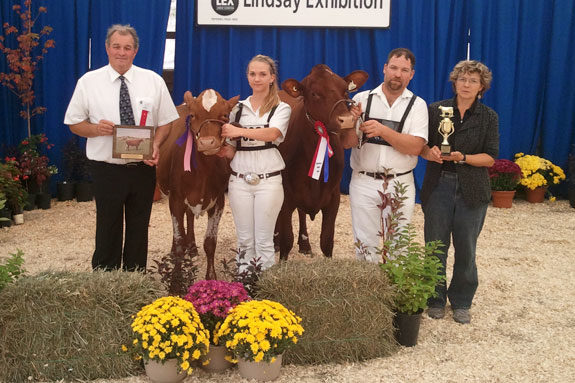In this vibrant image, likely taken at a state fair or farming competition, four individuals proudly present their award-winning cows against a backdrop of blue curtains and a partially visible sign. The scene is adorned with hay bales and pots of yellow and pink flowers, adding a rustic charm. 

On the far left stands an older man with short gray hair, dressed sharply in a white shirt and blue tie with black pants. He is happily holding a picture of a cow. Next to him, a brown cow with a white head prominently displays its medal and ribbon. A young blonde woman stands beside the cow; she is dressed in an all-white outfit with a black belt, a number partially covered on her chest. The next cow, completely brown and adorned with a red, blue, and white ribbon and medal, is held by a Caucasian man of heavier build wearing a similar all-white attire. He has brown hair and also sports a number and sign around his neck. On the far right, a middle-aged woman with short hair dressed in a green top and blue jeans smilingly holds a gold trophy. All individuals and animals are facing the camera, capturing a joyful moment of achievement in this detailed and lively scene.